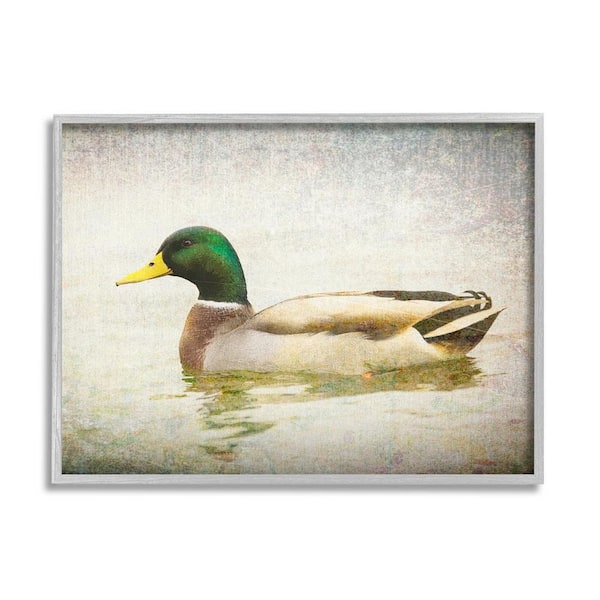This is a detailed, framed illustration of a mallard duck, set against a gradient background that transitions from dark gray to white at the top. The image captures a side view of the mallard, whose vibrant emerald green head and yellow bill contrast strikingly with its more muted body feathers of tans, browns, and creams. The duck floats serenely in the water, its reflection faintly visible, hinting at a greenish tinge in the water. Below the green head, a distinctive white ring encircles its neck, followed by a gray patch and further down, darker brown tail feathers. The scene is enclosed within a thin, white frame that complements the artwork's tranquil, somewhat faded aesthetic.